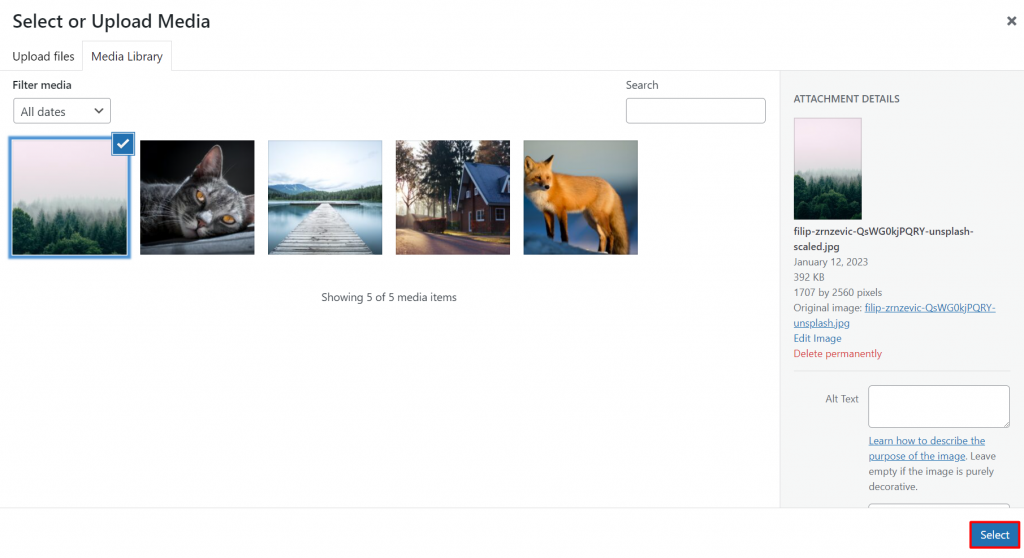The screenshot captures a media upload interface on a website, featuring a clean white background with various elements in black text and lines. On the left side, the interface prompts the user with options to "Select or Upload Media." To the right side of this prompt, there's a black 'X' for closing the window. Below the prompt, black text instructs the user to either "Upload Files or Use the Media Library."

Enclosed within a very thin black rectangular outline extending from the left to the right, there's another section. This section features a "Filter Media" option, next to which is a small black square with the text "All Dates" and a black down arrow indicating a drop-down menu.

Displayed below these options are five images. The first image, highlighted in white and marked with a blue square containing a white checkmark in its upper left corner, depicts a lush, green forest. Next to this image, there are photos of a cat lying down and staring at the camera, a dock on a serene lake with a cabin nestled in the forest, and a red fox sitting on snow.

Below these images, text indicates "Showing 505 Media Images." On the right-hand side, there is a detailed view within a gray box labeled "Attachment Details," showing information about the highlighted forest image. This includes the file name, JPEG format, date (January 12, 2013), file size (3.3, 92 KB), dimensions (1706 x 2560 pixels), and the original file image. There is also a blue underlined website link and an option to "Delete Permanently." Additionally, there's a section for adding alt text to describe the image better.

At the bottom right corner of the interface, there's a blue box with the white text "Select", completing the media upload interface.